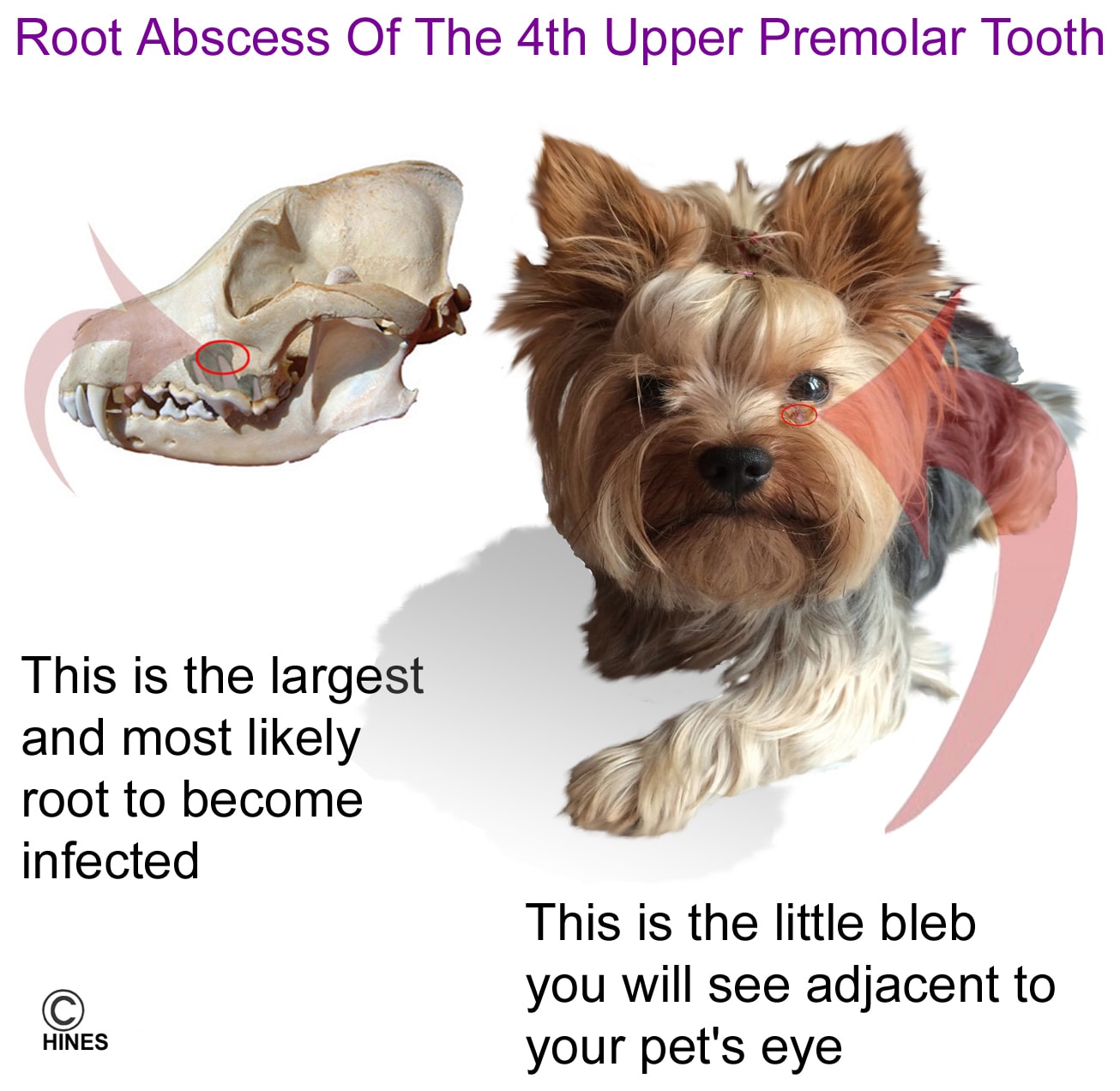The infographic illustrates a veterinary medical issue focusing on root abscess of the fourth upper premolar tooth in dogs. Centered on a white background, the right side of the image prominently features a small dog with yellow fur on its face, black eyes, and brown fur on its outward-pointing ears. The dog's front paw, covered in yellow fur, faces down towards the left. Notably, a large red arrow points to a small red circle situated just below the dog's eye, indicating the external location of the abscess.

On the left side of the infographic, there is a depiction of a dog's skull with another large red arrow pointing to a small red circle, highlighting the internal position of the affected tooth within the mouth. The top of the image is labeled in bold purple text: "Root Abscess of the Fourth Upper Premolar Tooth."

The bottom left of the diagram reads, "This is the largest and most likely route to become infected," while the bottom right annotation states, "This is the little bleb you will see adjacent to your pet's eye." A Heinz logo accompanied by a copyright symbol appears in the bottom left corner, signifying the source or sponsorship of the infographic. 

Overall, the infographic combines detailed illustrations and informative text to educate pet owners about this common dental issue in dogs.